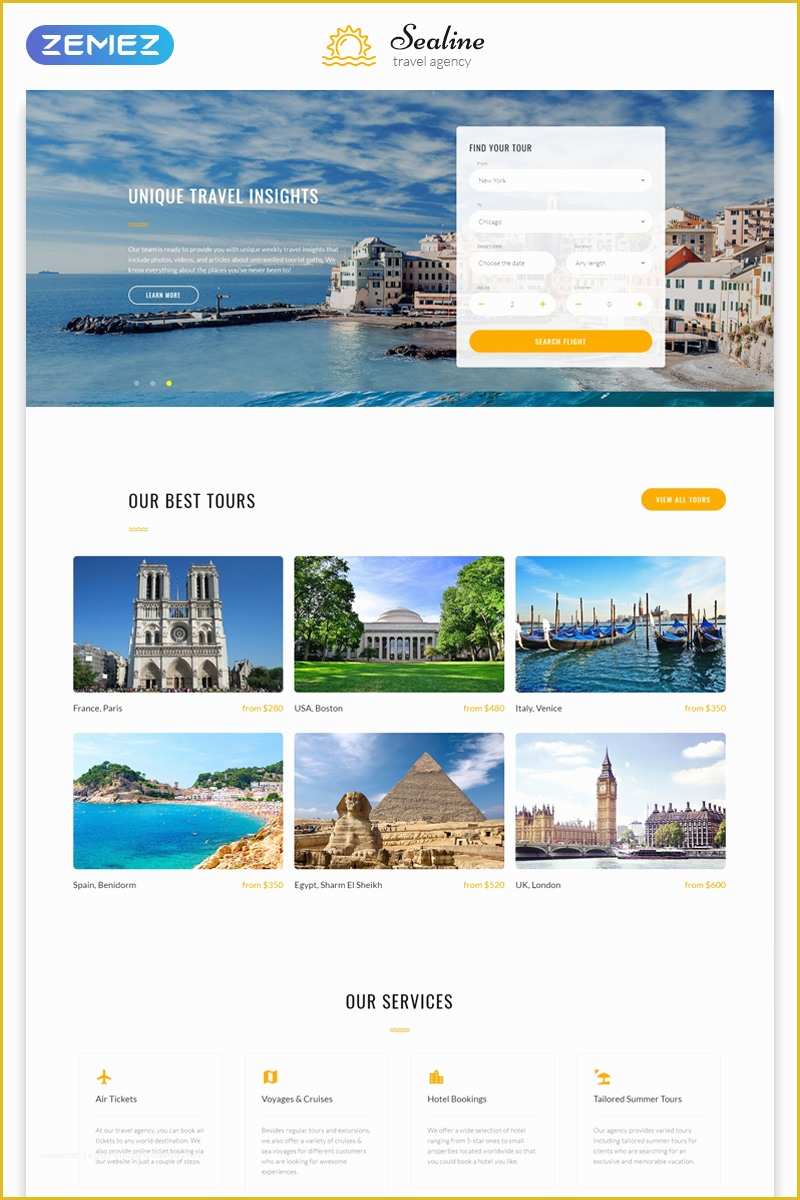The website header features a prominent blue oval button on the top left corner with the text "Zemez" inscribed in crisp white letters. Adjacent to it, there's a small yellow image of a sun with wavy stripes beneath it symbolizing water. Further to the right, centrally positioned at the top, is the website title "Sea Line" in bold black letters, with "Travel Agency" written below it in subtle gray text.

The main section of the page showcases a picturesque backdrop on the left side, depicting the serene ocean beneath a canopy of dark blue skies filled with fluffy white clouds. Contrastingly, the right side of the image is overlaid with a view of multiple tall brick buildings and an expanse of sandy beach. 

To the left of this image, the words "Unique Travel Insights" are prominently displayed. There is some smaller, unreadable text beneath this heading. On the right side, a booking interface titled "For Your Tour" allows users to input their departure date, return date, and the number of travelers. This section features an orange button labeled "Book" at the bottom.

Scrolling further down, a section titled "Our Best Tours" appears in bold black letters. Below this heading, six thumbnails showcase various travel destinations. The top-left thumbnail displays a grand building with a central circular clock, captioned "Paris." To its right, a thumbnail depicts an architecturally intricate building crowned with a dome, labeled "USA." Further right is an image of the ocean featuring long canoe-like boats, labeled "Venice."

On the bottom row, starting from the left, the first thumbnail presents a sandy beach with pockets of greenery and a portion of the ocean under a clear sky. Moving right, the next image showcases a blue sky above a pyramid and desert landscape. The final thumbnail on the right depicts a towering building with a pointed top, labeled "London."